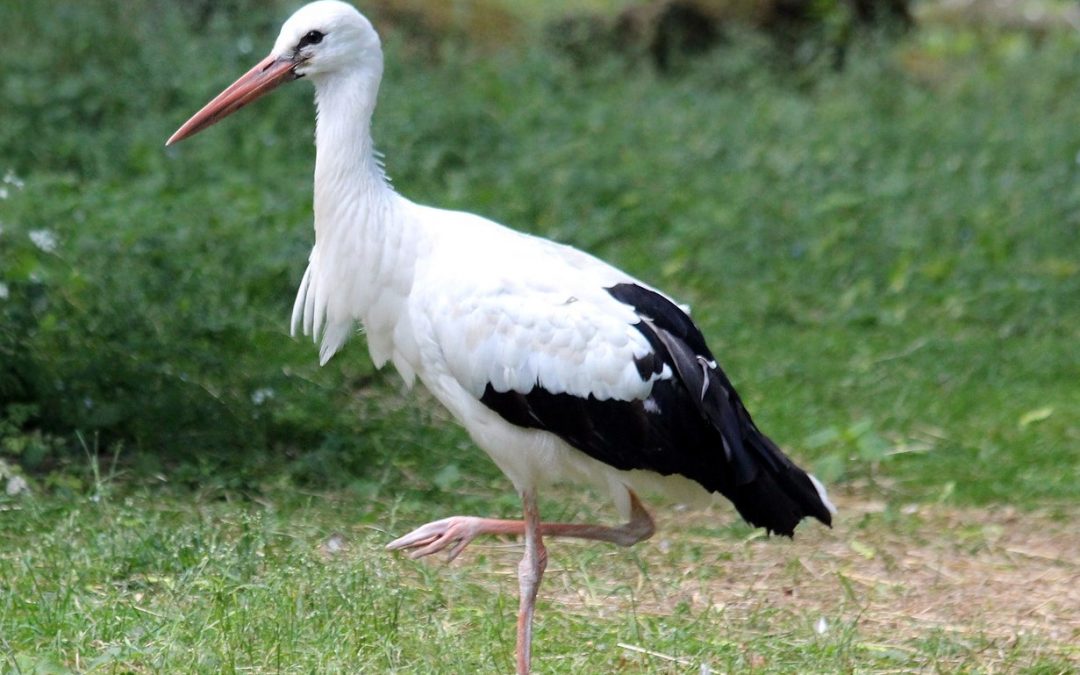The photograph captures a serene outdoor scene focused predominantly on nature, showcasing an elegant stork standing alone in a grassy environment. The image, taken in landscape orientation, features a tall, predominantly white stork slightly off-center to the left. The stork is facing left, offering a perfect profile view with its characteristic long, orange-pink beak and black eye. Its distinct plumage includes large white feathers on its chest and black tips on its wings and possibly its tail. The bird is notably standing on one leg, with the other leg tucked behind its body. Surrounding the stork, the ground is covered in varying shades of grass, transitioning from shorter green and brown grass in the foreground to taller, denser vegetation towards the background. The background is somewhat blurred, accentuating the stork as the central subject. The color palette of the scene comprises natural hues of brown, various shades of green, black, white, and the orange tones of the bird's beak and legs. The setting suggests a wild, untouched natural habitat, possibly an area frequented by a variety of bird species.